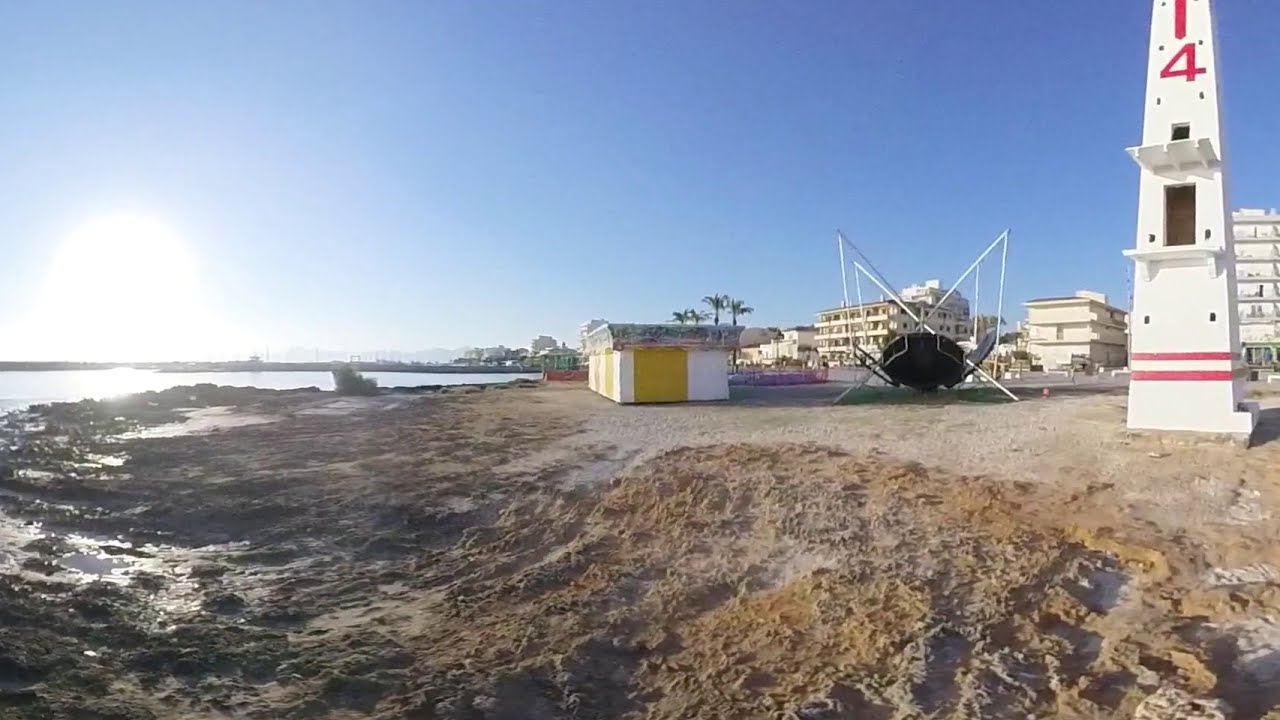The image depicts an outdoor coastal resort, likely in the Middle East, under a clear blue sky illuminated by a bright sun near the horizon on the top left. The scene includes a sandy beach with varying shades of sand, from darker, damp areas near the water to whiter, dryer sections. The left side features a tranquil sea. A prominent boat, black and seemingly permanent, rests on a stand on the beach. Near the center stands a squat white building with yellow doors, possibly a beach kiosk or changing huts. Dominating the right side is a white structure with two red stripes and the number 14 painted on it—likely a lighthouse or guard station. The background showcases several multi-story white buildings with balconies and numerous windows, suggesting they could be either apartments or a hotel. Palm trees are visible in the distance, adding to the tropical resort atmosphere.